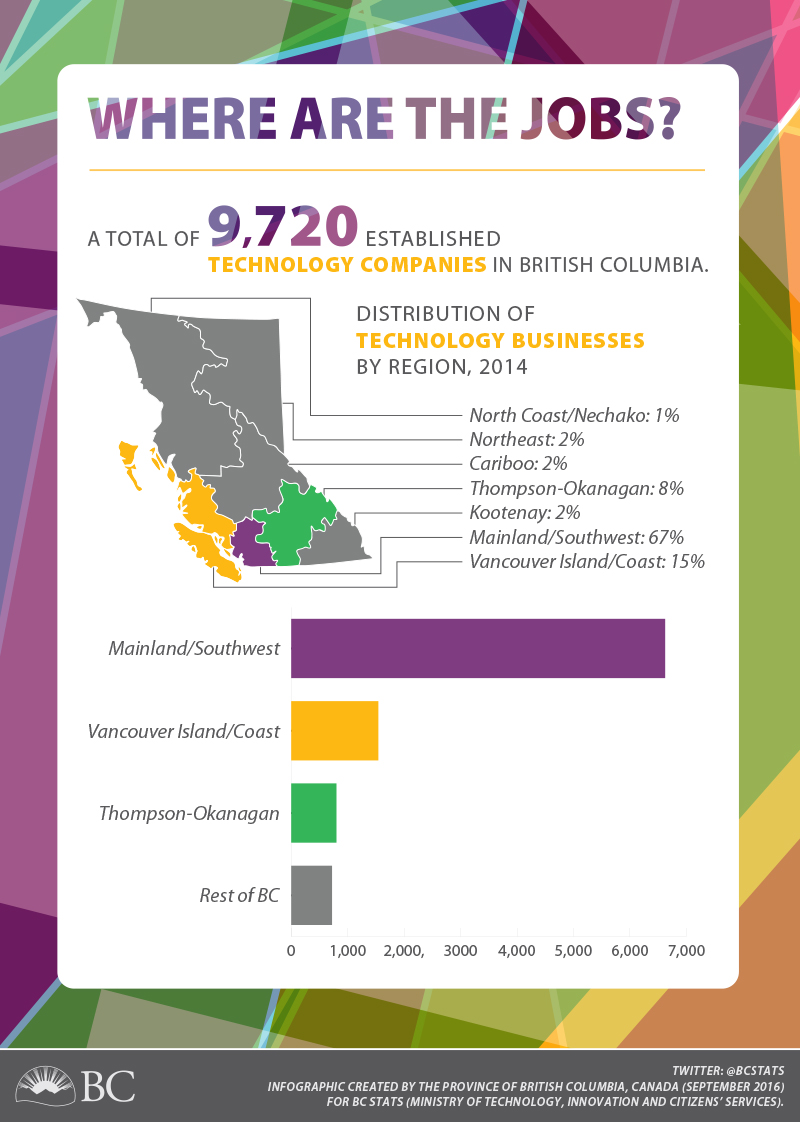This poster, set against a vibrant stained glass-like background featuring shades of pink, purple, green, yellow, and blue, displays an infographic about the distribution of technology companies in British Columbia as of 2014. The centerpiece is a white rectangle with detailed information. At the top, in bold purple capital letters, it reads "WHERE ARE THE JOBS?" Below a pale line, it states in gray letters that there are a total of 9,720 established technology companies, with the number emphasized in larger purple font.

On the left side of the white rectangle is a map of British Columbia, color-coded by region, showing the distribution of these companies. The regions and their respective percentages are: North Coast (1%), Northeast (2%), Caribou (2%), Thompson/Okanagan (8%), Kootenai (2%), Mainland/Southwest (67%), Vancouver Island/Coast (15%). A corresponding bar chart at the bottom right of the map visually represents these statistics, with Mainland/Southwest colored in purple, Vancouver Island/Coast in yellow, Thompson/Okanagan in green, and the rest of BC in gray. The x-axis of the chart ranges from 0 to 7,000, indicating the number of companies per region, with the Mainland/Southwest bar nearly reaching the 7,000 mark, Vancouver Island/Coast around 2,000, and the other regions significantly lower.

At the bottom of the poster, a gray strip contains the letters "BC" beside an emblem of a half-circle sunset and specifies that the infographic was created by the Province of British Columbia's Ministry of Technology, Innovation, and Citizen Services, specifically for BC Stats.